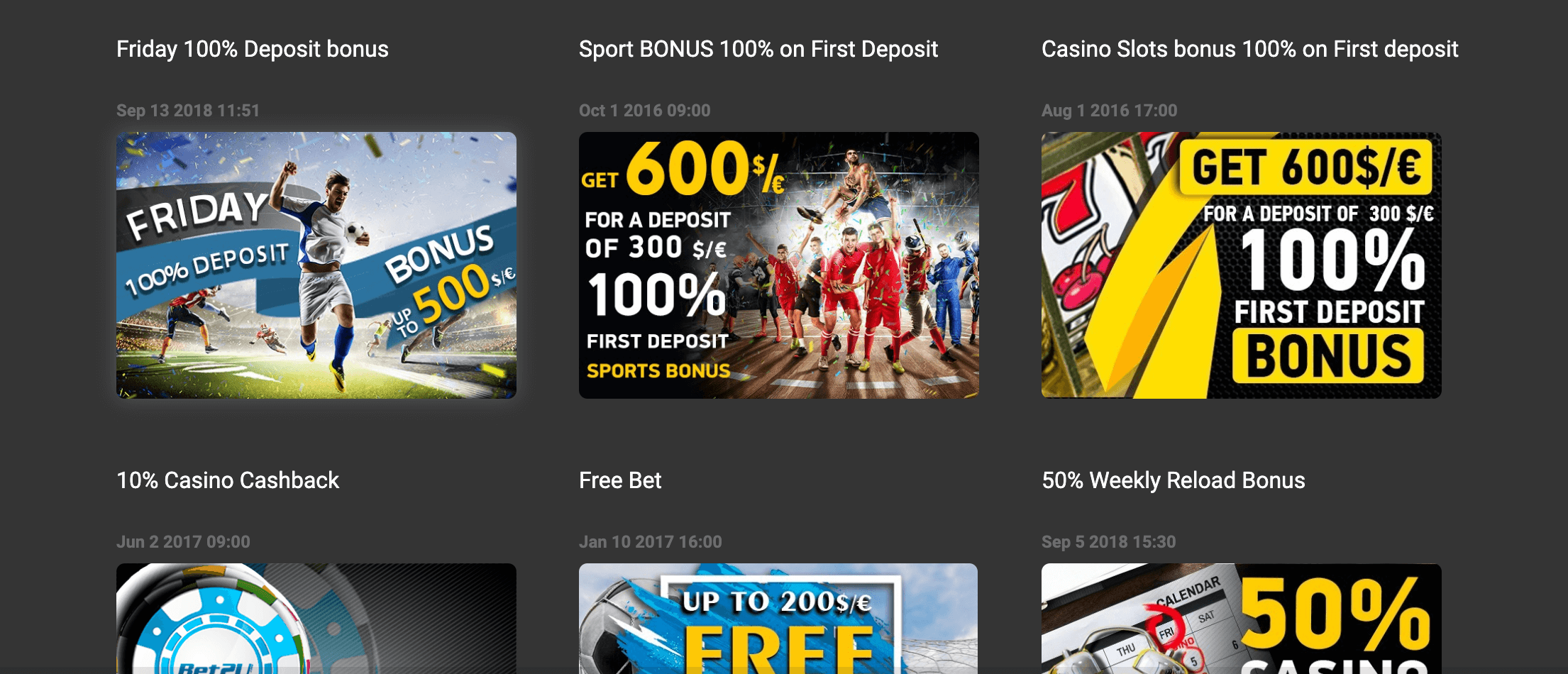The screenshot depicts a grey-background computer screen showcasing a series of online betting and gambling promotions, each detailed with specific offers and dates. At the top, the header prominently displays a "Friday 100% Deposit Bonus," dated September 13, 2008, at 11:51. The image includes a celebratory soccer player, indicative of a sports betting promotion that offers a 100% deposit bonus up to $500. 

Adjacent to this, a smaller caption "S/E" is barely noticeable. Below, there's a detailed description of a "Sports Bonus" offering a 100% match on the first deposit, with an example dated October 1, 2016, at 9:00 AM. It highlights a $600 reward for a $300 deposit, illustrated with images of two sports teams in red and blue jerseys, also in a celebratory stance.

The next segment promotes a "Casino Slots Bonus," also offering a 100% match on the first deposit, dated August 1, 2016, for $1,700. The visuals evoke a classic casino feel with symbols like red 7s and cherries. 

At the bottom, a series of promotions are listed from left to right:
1. A "10% Casino Cashback" offer dated June 2, 2017, at 9:00 AM, accompanied by an image of a blue and white casino token.
2. A "Free Bet" promotion dated January 10, 2017, at 4:00 PM, offering up to $200 free for sports betting, identifiable by a black and white soccer ball graphic.
3. A "50% Weekly Reload Bonus" dated September 5, 2018, at 3:30 PM, offering a 50% casino bonus. 

In the background, a calendar displaying the days Thursday, Friday, and Saturday is subtly visible, reinforcing the time-sensitive nature of these offers. The overall layout and content suggest an advertisement for various betting and casino sites, highlighting specific promotional deals and the corresponding dates.